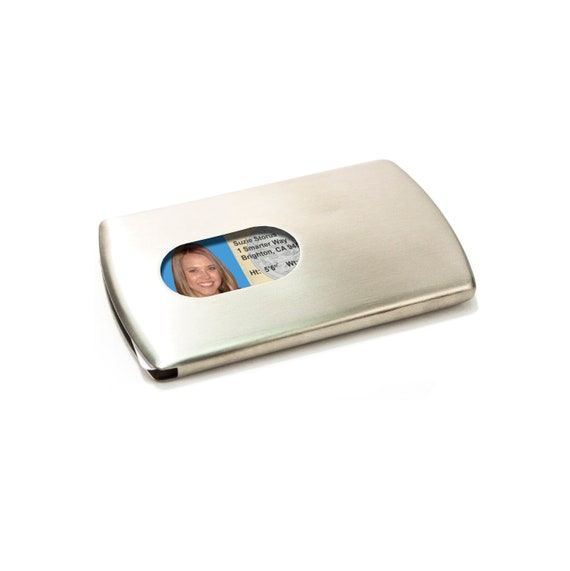This is an image of a small, modern, brushed stainless steel card holder wallet, designed to hold items such as a driver's license, credit cards, and potentially small bills. The wallet, compact enough to fit in a pocket, features an oval cutout on the front, through which an ID can be seen. The ID inside, displayed for illustrative purposes, is of a woman with blonde hair, who is smiling broadly, her teeth visible. The ID details reveal her name as Suzy Storis, residing at One Smarter Way, Brighton, California, with a height of 5'8". The ID itself has a blue background, complementing the minimalist and sleek design of the wallet, which lies flat against a white surface. The wallet's simple, flat, and thin form factor emphasizes a minimalist, modern aesthetic.